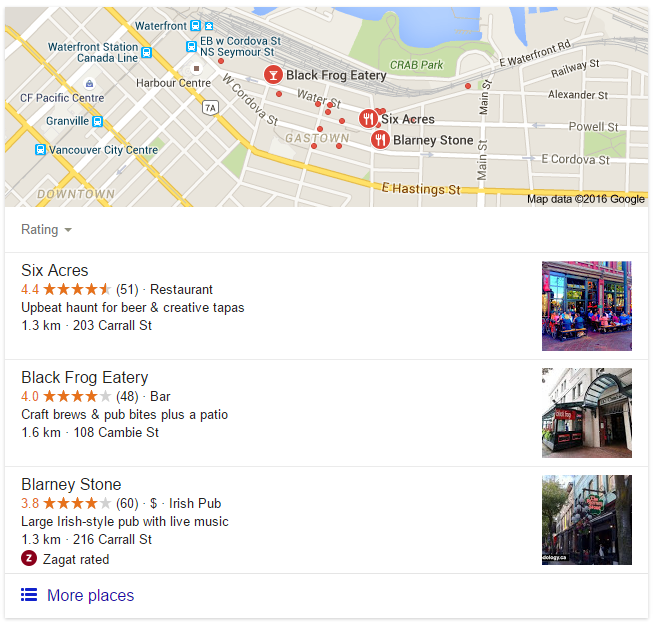The top portion of the image features a map highlighting the locations of three restaurants, each marked for easy identification. Below the map, detailed information and images of the three establishments are presented. 

On the left side, the restaurant "Six Acres" is showcased with a prominent image of its exterior and seating area. It boasts a rating of 4.4 stars based on 51 reviews. Described as an upbeat restaurant known for its beer selection and creative tapas, it is located 1.3 kilometers away at 203 Carroll Street.

On the right side, "Black Frog Eatery" is depicted through an exterior photograph showing patrons enjoying the patio seating. This bar holds a 4.0-star rating from 48 reviews and offers craft brews and pub bites. It is situated 1.6 kilometers away at 108 Cambie Street.

The last restaurant, "Blarney Stone," has a more budget-friendly $1 sign and is represented with images of its lively ambiance. This large Irish-style pub features live music and has received a 3.8-star rating from 60 reviews. It is conveniently located 1.3 kilometers away at 216 Carroll Street.

All three restaurants appear to be close to the waterfront, possibly situated in Vancouver City Center, Vancouver. At the bottom of the image, there is an aggregated section with three blue lines and a "More Places" button in blue, indicating additional restaurant options.